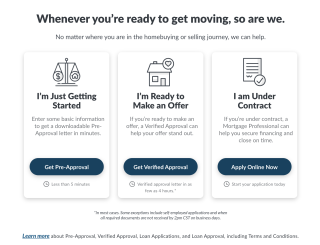Screenshot of a real estate website designed to assist home buyers. The interface features a clean, white background with primarily black text and dark blue buttons. At the top of the page, a prominent heading reads, "Whenever you're ready to get moving, so are we." Beneath this, a subheading reassures users, stating, "No matter where you are in the home buying or selling journey, we can help."

The visual is small, making some text difficult to discern, but it displays three horizontally aligned boxes, each representing a different stage in the home buying process. 

1. **Just Getting Started**: The first box features an icon of scales with a dollar sign on one side and a home on the other. It includes a brief description and a call-to-action button labeled "Get Pre-Approval."

2. **Ready to Make an Offer**: The second box showcases an icon of a home with a heart above it. It includes the message and a call-to-action button labeled "Get Verified Approval."

3. **Under Contract**: The third box has text indicating this stage, accompanied by an icon and a button labeled "Apply Online Now."

Each box provides a concise description under its respective icon, guiding users through their home buying journey.